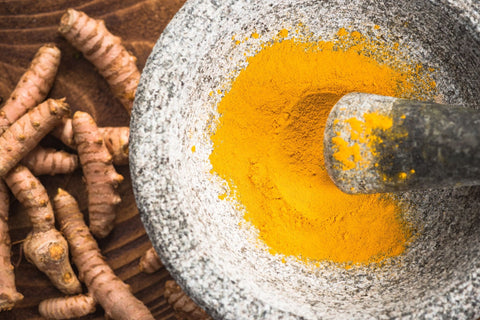The rectangular photograph features an up-close view of a mortar and pestle grinding what appears to be turmeric root into a fine powder. The mortar and pestle occupy the right two-thirds of the image, both predominantly gray with specks of black; however, the pestle has a more pronounced black handle. Inside the bowl of the mortar lies a vibrant yellow-orange powder, presumably ground from the turmeric roots visible on the left one-third of the image. These root-like, nubbed plants, bearing a strong resemblance to ginger, are scattered on a dark brown wooden surface with lighter wood grain highlights. The overall composition accentuates the transformation from whole turmeric roots to vividly colored, finely ground powder.